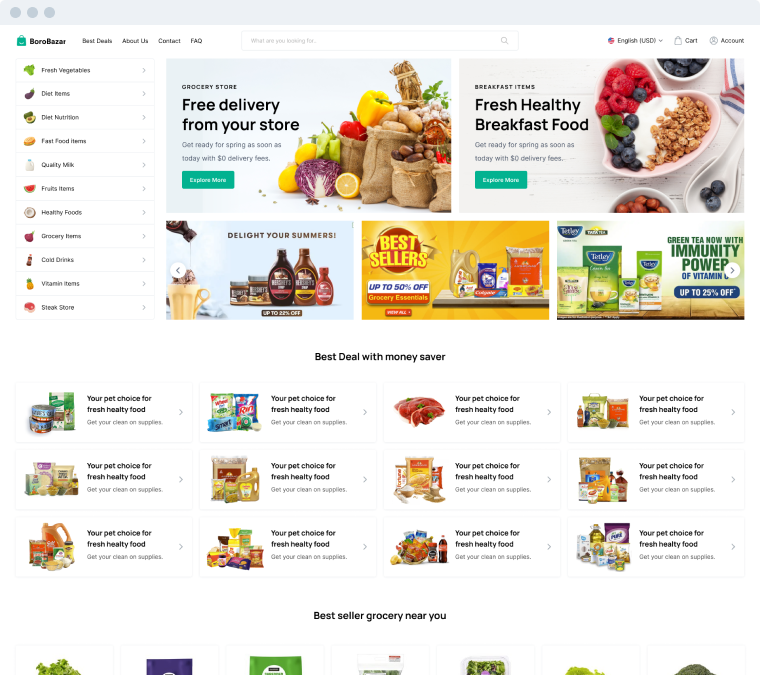Website Screenshot Description:

The screenshot captures the homepage of a website named "BORBAZAR." The name "BORBAZAR" is prominently displayed at the top of the page. Just below the website name, there is a navigation menu that includes the following tabs: "Best Deals," "About Us," "Contact," and "FAQ." To the right of the navigation menu, there is a search bar with the placeholder text "What are you looking for," followed by language selection "English," currency selection "USD," a "Cart" icon, and an "Account" option.

On the far left side of the page, there is a vertical menu listing various categories, which include: 
- Fresh Vegetables
- Diet Items
- Diet Nutrition
- Fast Food Items
- Quality Milk
- Fruits Items
- Healthy Foods
- Grocery Items
- Cold Drinks
- Vitamin Items
- Steak Store

To the right of this vertical menu, there is a large photograph featuring numerous bags filled with colorful produce atop a countertop. Overlay text on the image reads: "Free delivery from your store. Get ready for spring as soon as today with zero dollar delivery fees."

Next, there is an image showcasing a heart-shaped white bowl filled with raspberries, blueberries, yogurt, and granola, accompanied by the text: "Fresh healthy breakfast food. Get ready for spring as soon as today with zero dollar delivery fees."

Below this, an image depicts several bottles of Hershey's syrup and the accompanying caption states: "Delight your summers. Up to 22% off."

Adjacent to this is an image displaying various items on a shelf labeled: "Best sellers. Up to 50% off grocery essentials."

Further down, another image features numerous boxes of Tetley tea with the caption: "Green tea. Now with the immunity power of vitamin C. Up to 25% off."

Beneath these promotional images, there are sections with repeat text stating "Best deal with money saver," and "Your pet choice for fresh healthy food," repeated multiple times.

At the bottom of the screenshot, partly visible, it reads: "Best seller grocery near you," but the accompanying images are cut off at the bottom of the screenshot.